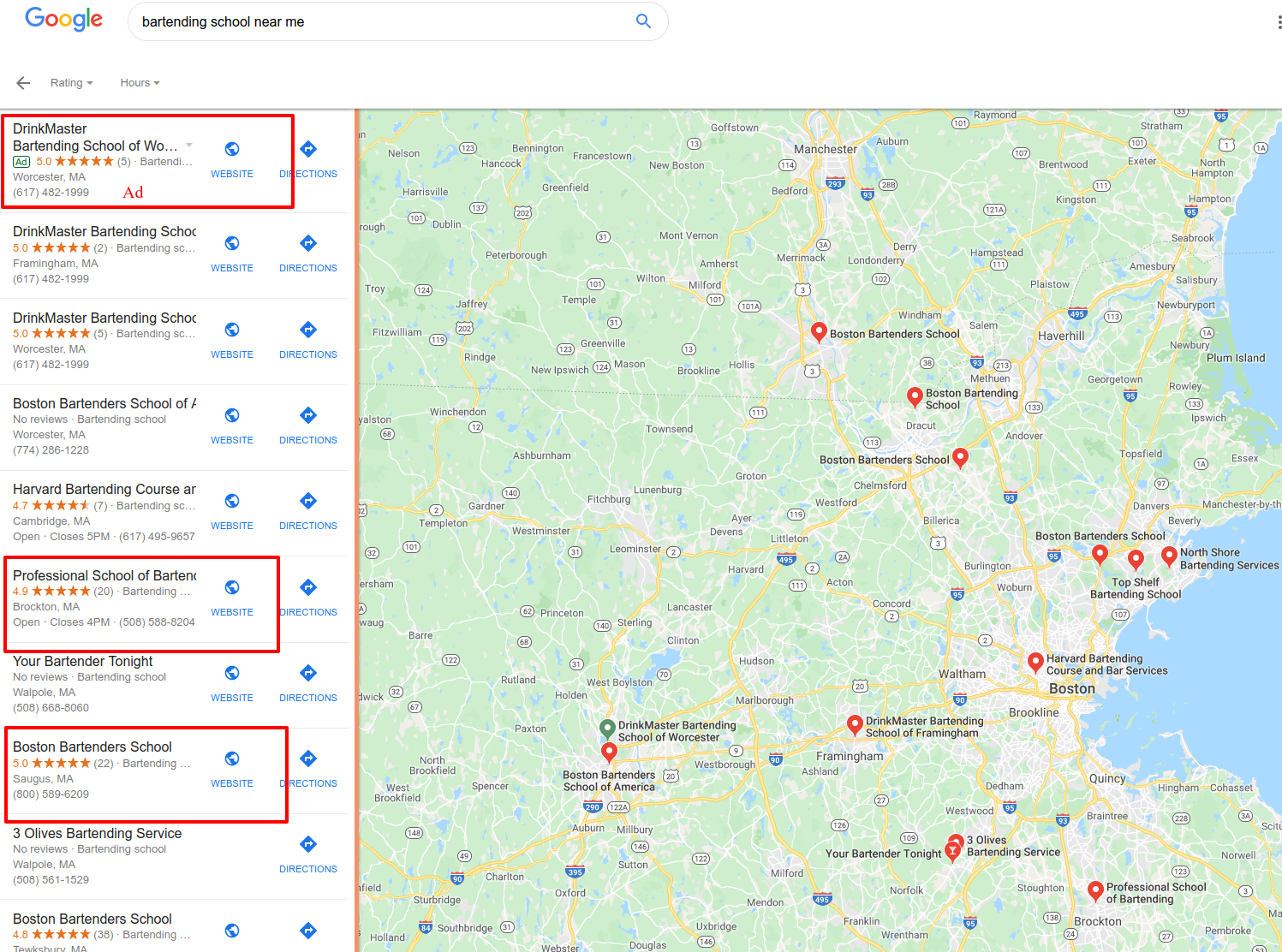This image is a screenshot from a Google Maps search for "bartending school near me." The right two-thirds of the screen features a detailed map of the Greater Boston area highlighting various bartending schools with red location markers. The areas visible on the map stretch from Boston, Brookline, and Brockton in Massachusetts to Troy and Manchester in New Hampshire, extending to West Brookfield and Rentham, and further reaching up to North Hampton and Hampton Beach.

The left-hand one-third of the screen presents a list of bartending schools available in the area. The schools listed, some of which are marked with red highlights, include:

1. DrinkMaster Bartending School of W.O. of Worcester
2. DrinkMaster Bartending School
3. DrinkMaster Bartending School
4. Boston Bartender School
5. Harvard Bartending Course
6. Professional School of Bartenders 
7. You’re a Bartender Tonight 
8. Boston Bartender School 
9. Three Olives Bartending School 
10. Boston Bartending School  

The red highlights around the names indicate selected or highly-rated options such as DrinkMaster Bartending School of W.O. of Worcester, Professional School of Bartenders, and Boston Bartender School.